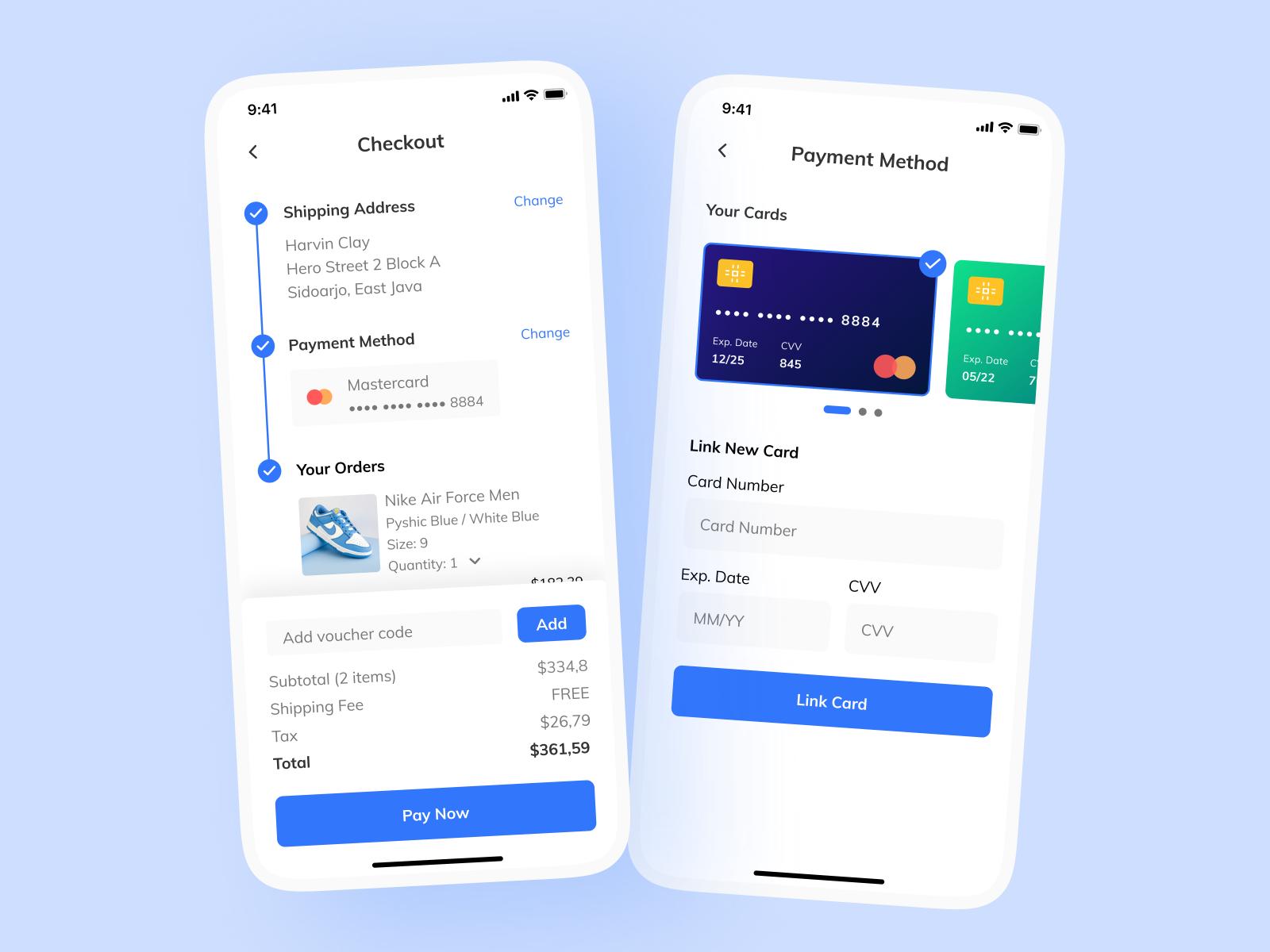In the image, there are two cell phones displayed against a blue background.

**Left Phone:**
- Screen Background: White
- Time Display: 9:41
- Status Bar: Full Wi-Fi and battery
- Checkout Screen Elements:
  - Title "Checkout" in black at the top
  - Shipping Address: "Horn Harvin, Clay Hero Street, 2 Block A, Sidarora, Joes Java"
  - "Change" link in blue next to the shipping address
  - Payment Method Section:
    - "Change" link in blue
    - Mastercard ending in 8884
  - Order Details:
    - Product: "Nike Air Force Men's"
    - Color: "Psych Blue/White/Blue"
    - Size: "9"
    - Quantity: "1"
  - Add Voucher Code Section:
    - "Add" button in blue
  - Summary:
    - Subtotal for Two Items: "$334.80"
    - Shipping: "Free"
    - Tax: "$26.79"
    - Total: "$361.59"
  - "Pay Now" button in blue at the bottom

**Right Phone:**
- Payment Method Screen Elements:
  - Title: "Payment Method"
  - Available Cards:
    - Mastercard ending in 8884, marked as blue and checked
  - Card Details:
    - Expiration Date: "12/25"
    - CVV: "845"
  - Options to:
    - "Add New Link"
    - "New Card"
    - "Card Number" input field at the bottom

This descriptive outline captures the intricate details and layout of the content shown on both cell phone screens.